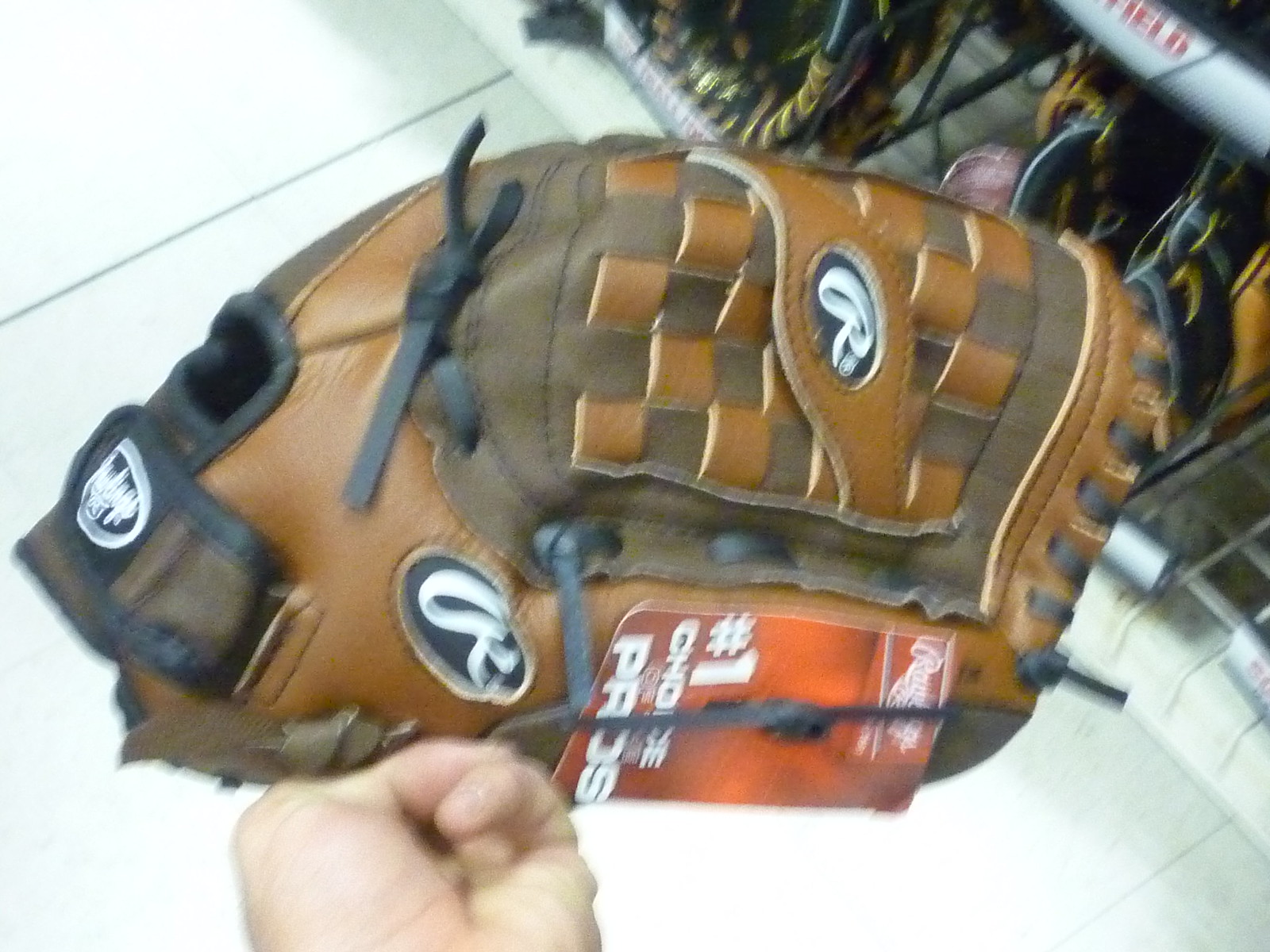This close-up photograph taken indoors captures a detailed view of a baseball glove being held by what appears to be a Caucasian male hand. The baseball glove, made of rich, natural British tan leather with chocolate leather accents and black laces, prominently features a white logo in the shape of a big 'R' enclosed in a black circle, indicating it is a Rawlings glove. A red tag on the glove reads "Rawlings, number one choice pros." The glove also has small, white-inscribed circles with the letter 'R' on them. In the background, the white tile floor is visible. To the upper right, a shelf displays other baseball gloves, and part of a white and red baseball bat with "Field" written on it can be seen, lined with a thin blue stripe. The image suggests the scene is set in a store, where someone is likely selecting a glove. The photograph appears slightly blurry, especially around the edges.